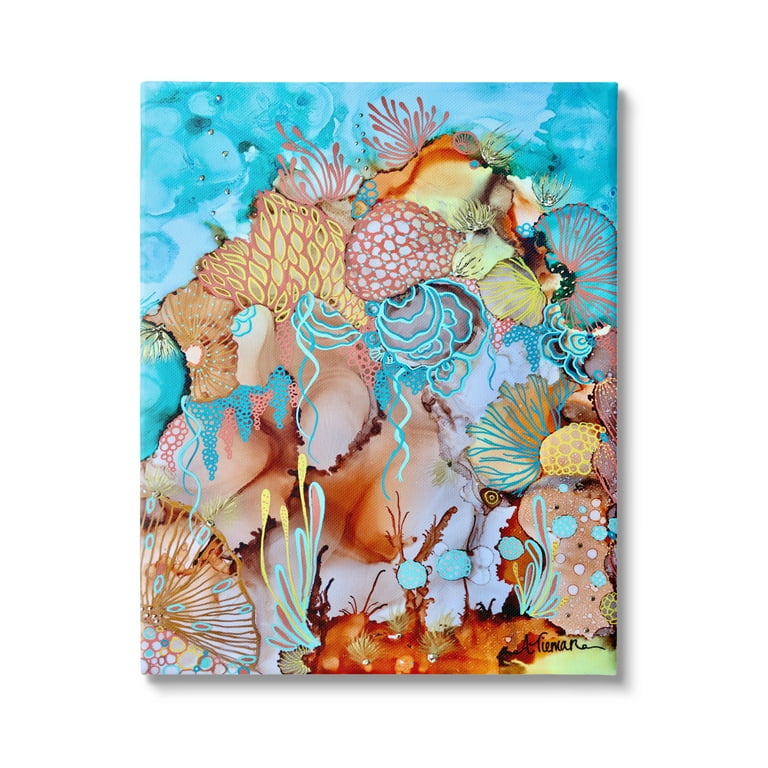This image portrays an abstract underwater scene, resembling a vibrant coral reef, meticulously painted in a watercolor style. The dominant background is a light blue turquoise, reminiscent of the sea. The foreground is a vibrant conglomeration of corals, sea anemones, and other marine organisms depicted in a broad palette of vivid colors. Among the detailed features, there are bright pink sea anemones at the top, and a mix of yellow, pink, brown, and blue corals. The scene includes tendrils of blue interweaving through the corals and pink sea cucumbers positioned to the right side. Blue bubbles add to the underwater effect. Interspersed are various coral-like structures in nude blush shades, some abstract copper and brown tones, and elements resembling seaweed and shells. Although some shapes are abstract and open to interpretation, they contribute to the overall vibrant and lively underwater aesthetic. The artist’s signature can be spotted in the bottom right corner, completing the intricate underwater tableau.